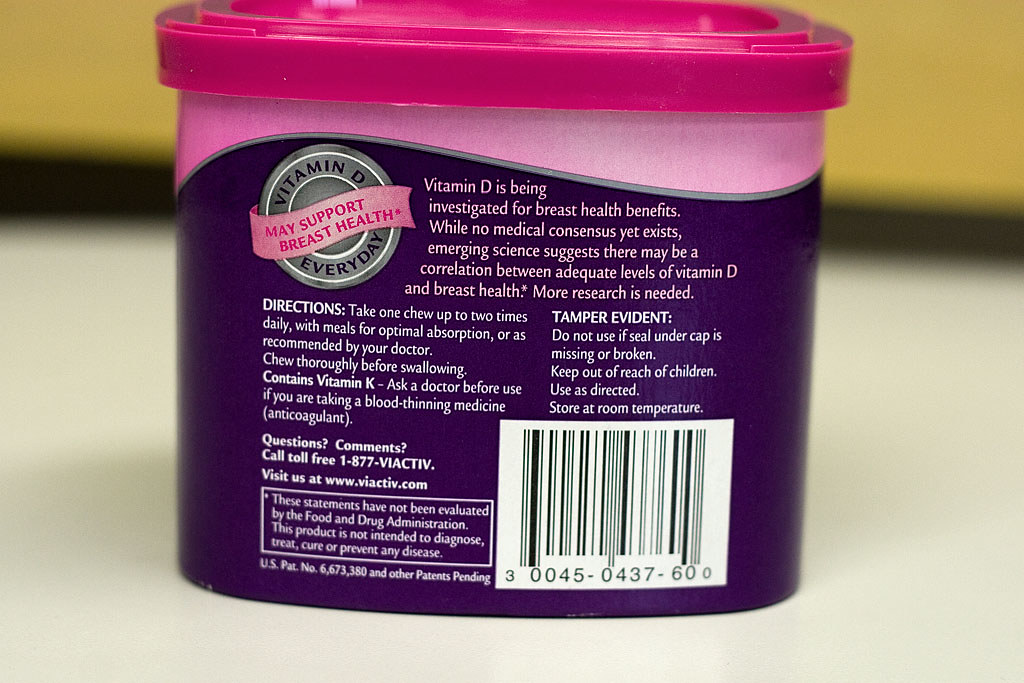The image showcases a tub-like product prominently displayed on a clean, white platform. The product features a visible label on its side. In the background, a mix of out-of-focus yellow and black elements add depth but do not distract from the main focus. On the top left of the image, text reads, "Vitamin D may support breast health every day." Adjacent to this text, a more detailed note elaborates, "Vitamin D is being investigated for breast health benefits. While no medical consensus yet exists, emerging science suggests there may be a correlation between adequate levels of Vitamin D and breast health. Asterisk. More research is needed." The composition highlights the product while subtly emphasizing the potential health benefits linked to Vitamin D.